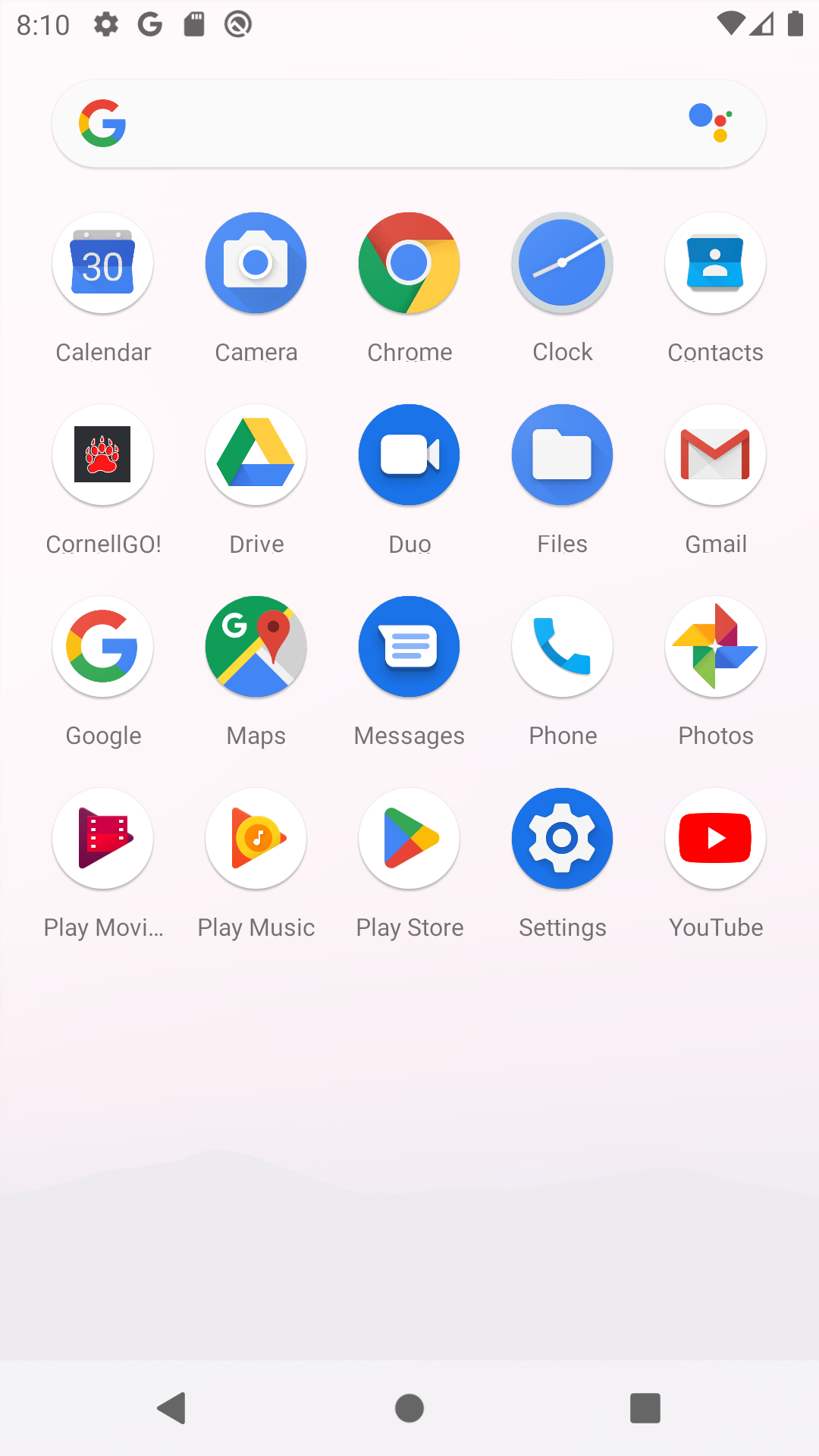Here is a cleaned-up and detailed caption for the provided image description:

---

This screenshot captures the home screen of an Android device, showcasing a neatly organized grid of app icons against a plain white background. The Google search bar, featuring the Google Assistant logo, is prominently displayed at the top, indicating that this is not the app drawer but the home screen. 

The layout includes the following apps:
- Top row: Calendar, Camera, Google Chrome, Clock, Contacts
- Second row: Cornell (unknown app), Google Drive, Google Duo, Files, Gmail 
- Third row: Google app, Google Maps, Messages, Phone, Google Photos 
- Fourth row: Google Play Movies, Google Play Music, Google Play Store, Settings (gear icon), YouTube (red icon)

The standard notification icons are visible at the top of the screen, and the familiar navigation buttons are located at the bottom.